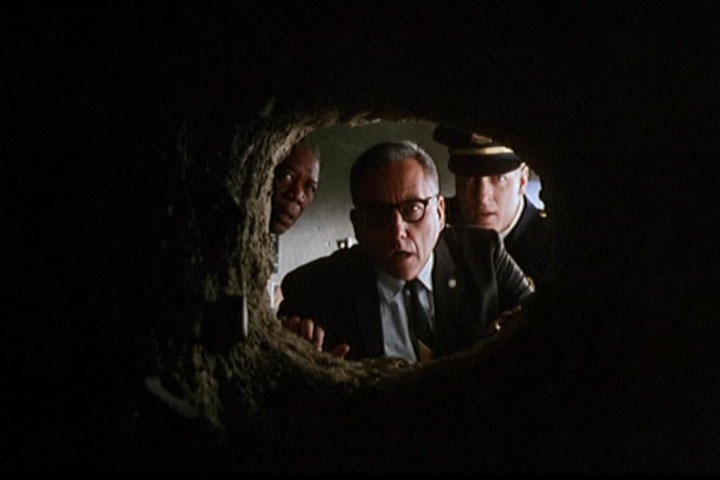In this scene from the movie "The Shawshank Redemption," the camera captures an intense moment of realization. On the left stands Morgan Freeman, distinguished in a black suit, white collared shirt, and black tie, with glasses framing his face. His expression is one of profound surprise. Next to him, at the center, is the warden, dressed in a gray suit and a gray and yellow tie, also wearing glasses. His hair is gray, and he too looks astonished as he peers into a tunnel carved into what appears to be a vault. The right side of the scene features a policeman in uniform, complete with a black hat, who shares in the collective shock. The setting behind them is dimly lit, with light filtering through windows, casting shadows on the gray walls. The tunnel in question is just large enough for a man to crawl through, with its entrance shrouded in darkness that deepens as it recedes from the observers' view. The entire scene radiates tension and disbelief, capturing a pivotal moment in the story.